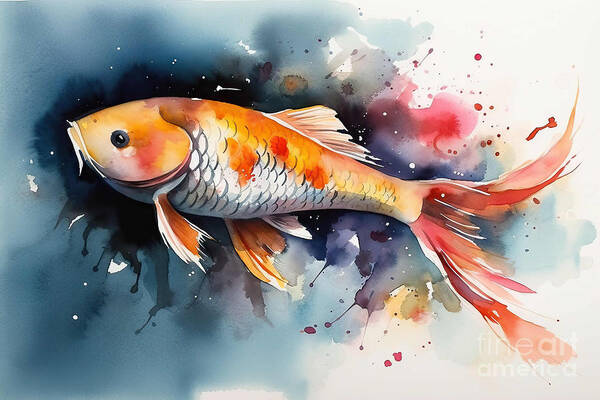This image depicts a vibrant fish, most closely resembling a goldfish, rendered in a watercolor or pen and ink style. The composition is horizontal and rectangular, with the fish positioned centrally, moving from left to right. The fish boasts a striking coloration: its head and back are vivid orange, accented with red markings behind its black, camera-facing eye. The belly transitions to white, and the tail appears frayed, blending shades of red, pink, and light orange. Some fins mirror this orange hue.

The background exhibits a striking contrast, dominated by hues of black to blue on the right side, suggesting an unusual setting that doesn't mimic typical aquatic environments. This area is punctuated by splatters and dots reminiscent of spilled ink or paint, incorporating additional colors like red, purple, and yellow. Flecks of white and lighter shades are also present, countering the dominant darker tones. Notably, a watermark in the lower right corner reads "Fine Art America," identifying the artwork's origin.